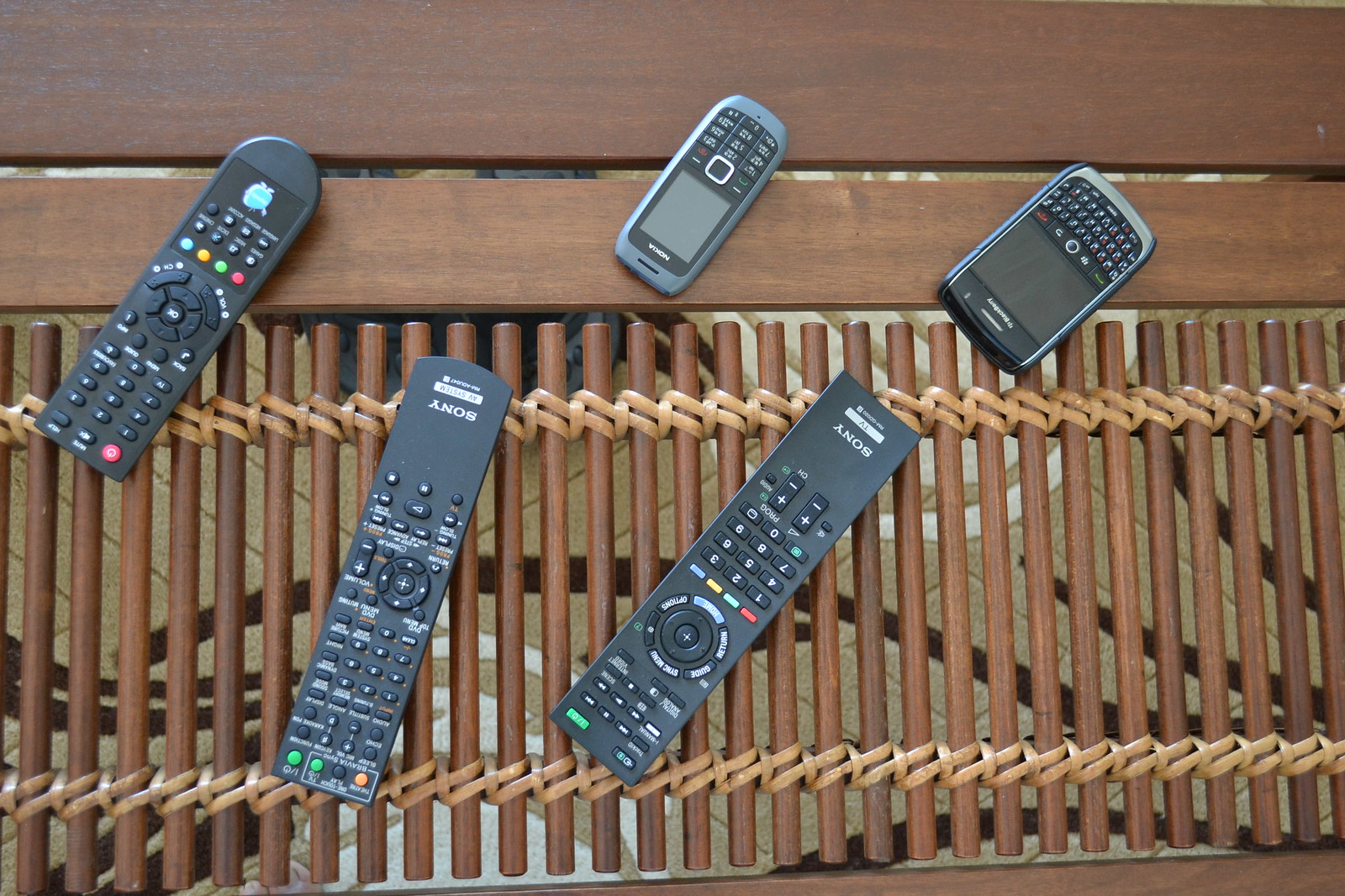This is a photograph taken from above of a medium-brown wooden surface, likely either a coffee table or a park bench. The image shows five distinct electronic devices arrayed on the wood, all primarily black in color. 

Starting from the upper left, there is a rectangular remote with rounded edges next to two Sony remotes, both designed for receivers, with one having more buttons than the other. To the right of the rightmost Sony remote is a gray Nokia cell phone, positioned in the center top of the image. Above, slightly to the right of the Nokia, is a white and black Blackberry-like device. 

The remotes and devices are scattered across the surface all pointing roughly towards the 7 o'clock direction. The wooden platform they rest on features vertical dowels tied together at the top and bottom with twine, creating a natural backdrop for the array of electronics.